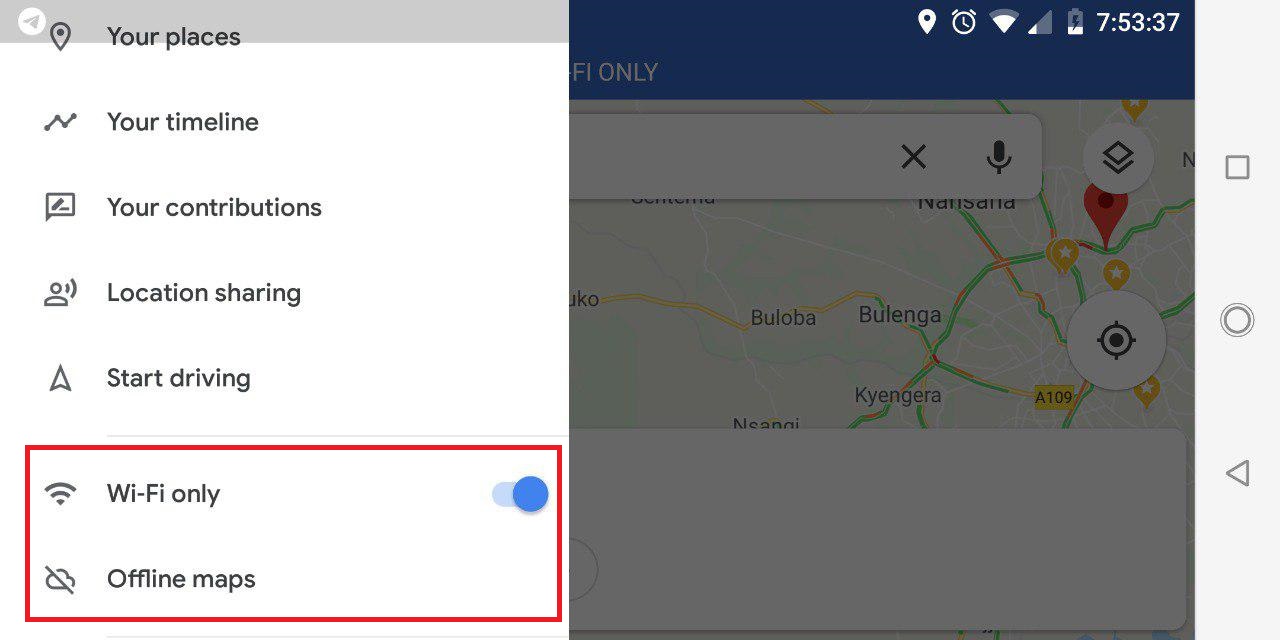The image is a screenshot of a mobile device displaying a navigation app. The top-right corner of the screen shows various status icons including the time (7:53:07), battery charging icon, network signal indicator, Wi-Fi signal indicator, alarm active icon, and location icon. To the left, a menu is visible, listing items such as "Your places," "Your timeline," "Your contributions," "Location sharing," "Start driving," "Wi-Fi only" (which is checked), and "Offline maps." "Wi-Fi only" and "Offline maps" are highlighted with a red bar. In the background, a map pane displays several locations, including Buluba, Bulenga, and Kyengera.